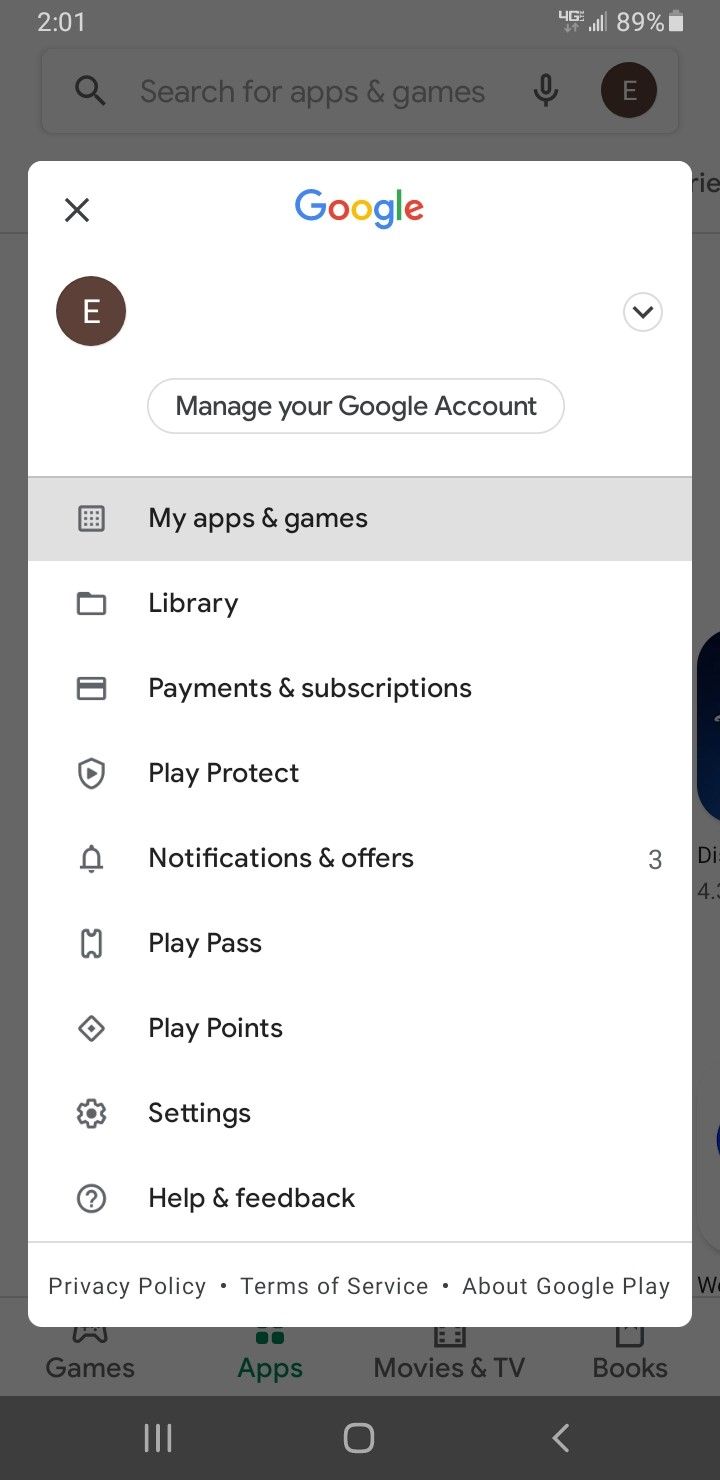This screenshot captures the screen of a cell phone, focusing solely on the display without revealing the phone's exterior or bezel. The background is a neutral grey. 

At the very top, the status bar indicates the time as 2:01. To the right of the time, it shows the device's connectivity status with a "4G" label and about 4 or 5 signal bars. The battery life is displayed at 89%, accompanied by a battery icon.

Just below the status bar is a search bar for apps and games, which includes a microphone icon and a circular icon with an "E" in it.

Beneath the search bar is a white rectangular section featuring the "Google" logo, spelled out in its distinctive blue, red, yellow, blue, green, and red colors. Under the Google logo is another circular icon with an "E".

Below the logo, a title reads "Manage Your Google Account." Featured are the following options:

1. My Apps and Games (highlighted)
2. Library
3. Payments and Subscriptions
4. Play Protect
5. Notifications and Offers (with a "3" indicating the number of notifications)
6. Play Pass
7. Play Points
8. Settings
9. Help and Feedback

At the bottom of the screen, three links are listed: Privacy Policy, Terms of Service, and About Google Play.